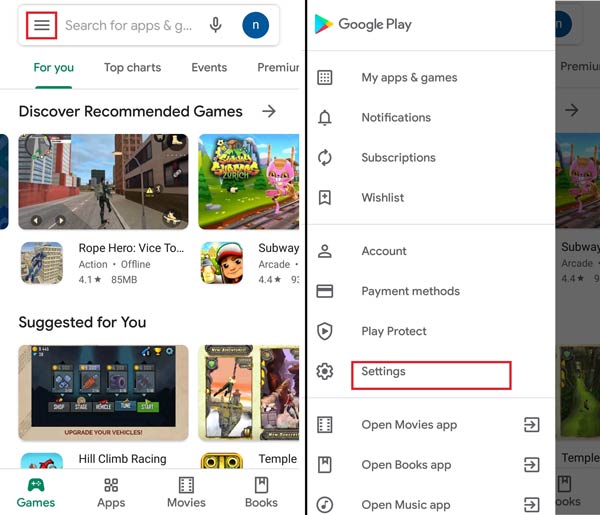In this image, we see a screenshot with a predominantly white background, except for a light gray border on the right. In the upper left corner, there's a white search bar that reads "Search for apps and G". Adjacent to the search bar, on its left, is a menu icon outlined in a red border, represented by three horizontal lines. In the upper right corner, there's a user icon represented by the letter "N" inside a blue circle.

Below the search bar, a horizontal menu spans the image. The first item is "For you" in green text with an underline, indicating an active link. Following it, in sequence, are "Top charts", "Events", and "Premium". 

The main section below the menu begins with the heading "Discover recommended games" in bold black text. To the right of this heading is a small arrow, likely for navigation.

In the right column, the first item is the "Google Play" heading, followed by a list of options beneath it. These options are: "My apps and games", "Notifications", "Subscriptions", "Wishlist", "Account", "Payment methods", "Play Protect", and "Settings", which is also outlined in a red border. Below these, there are options to "Open movies app", "Open books app", and lastly, "Open music app".